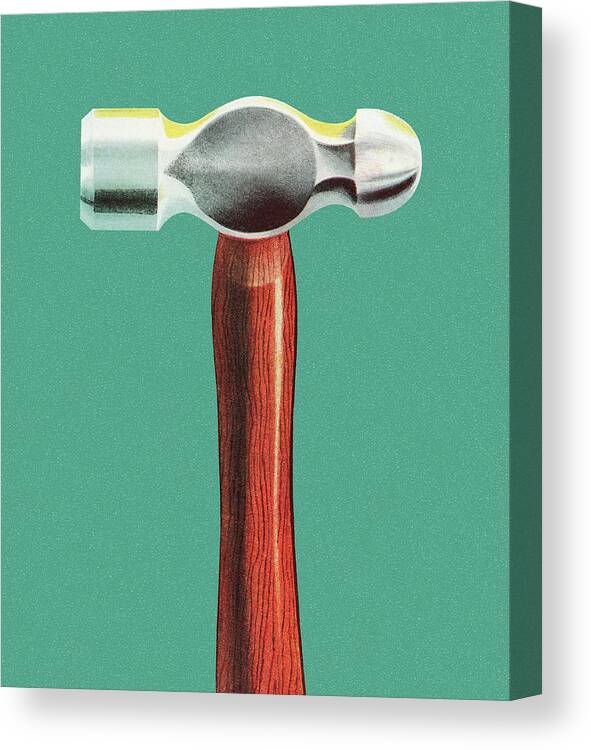This image features a detailed painting of a ball-peen hammer on a green canvas which is mounted on a rectangular frame, partly visible at the top, right, and bottom with a thicker white border surrounding these sides. The canvas, medium green in color, stretches around the entire inch-deep frame, though the left side of the frame is not visible, appearing cut off. The hammer depicted has a prominent brown wooden handle with vertical dark grain, extending vertically from the bottom to about three-quarters up the canvas. A streak of lighter color runs vertically along the handle, with additional subtle shadows creating depth. Atop the handle is the metallic hammerhead, featuring a cylindrical shape on the left and a hemispherical, dome-like shape on the right, with a central circular joint connecting it to the handle. The background remains completely white, emphasizing the hammer as the central subject of the painting.